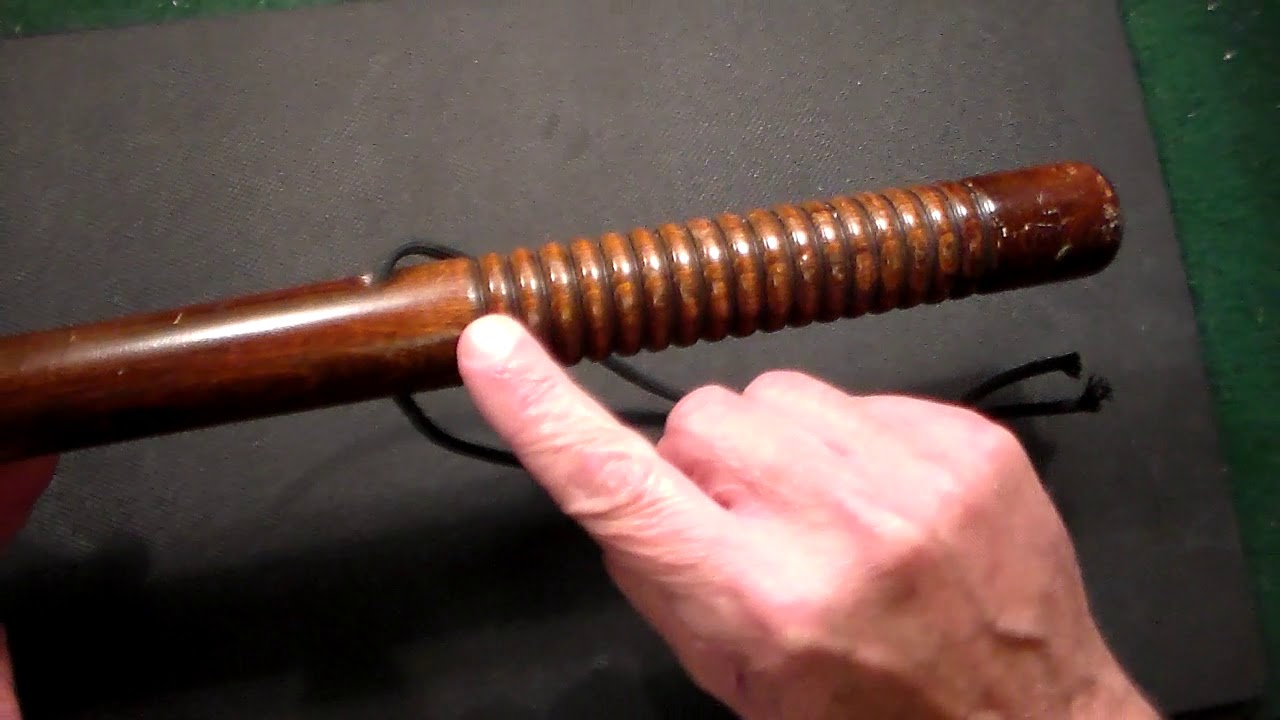The image depicts a close-up view of a brown billy club with a rich cherry wood appearance, showcasing a textured handle with spiral-shaped ridges. The handle has small slits and cuts, indicating that it has been used and is not brand new. A black cord is threaded through a hole in the handle, with its loose ends visible, suggesting it can be hung. The focal point of the image is a light-skinned man's right hand, seen from the wrist up, pointing specifically at one of the darker brown circular patterns on the grip portion of the billy club. The handle is resting on or slightly above a green table, with a black piece of cardboard or thin stone beneath it. The man's left hand is partially visible, with just one finger peeking into the frame.